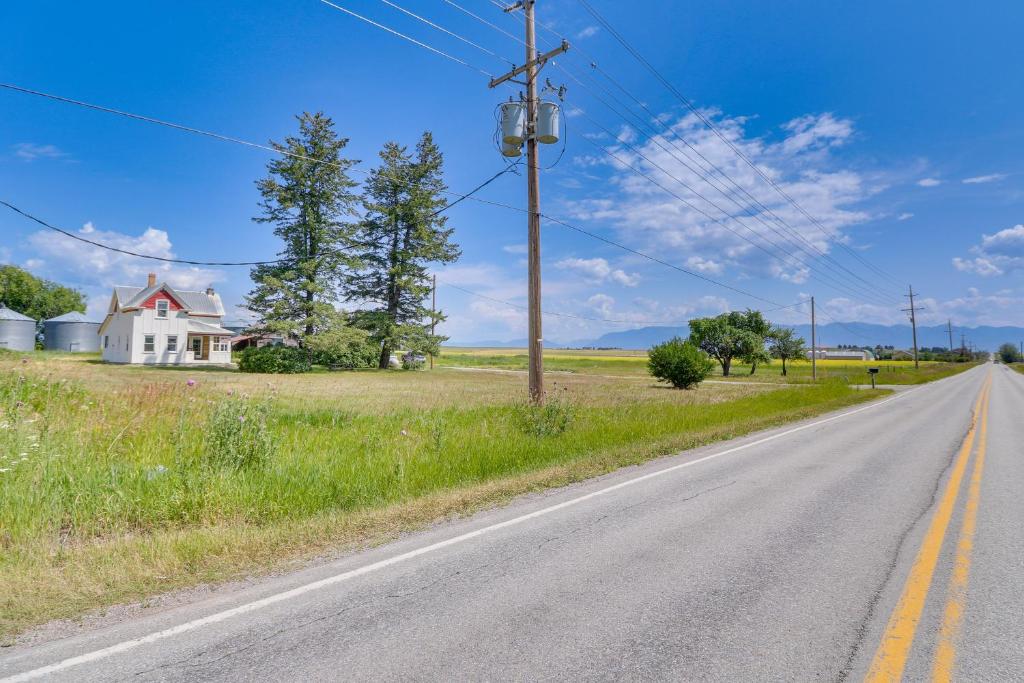This vibrant, square, full-color photograph captures a tranquil rural scene on a mostly sunny day, bathed in natural light. Dominating the image on the left side is a charming white two-story farmhouse with a gray metal roof and red trim around the second-story window. The house features a central entranceway, possibly leading to a small porch, and is flanked by two large deciduous trees, likely oaks, along with a bush and a smaller tree resembling a fruit tree. 

In the foreground, a light gray asphalt two-lane road with yellow no-passing lines stretches diagonally from the lower left to the center right of the image, framed by white edge lines near grassy ditches. The road appears to extend endlessly into the distance, where another property is faintly visible. A wooden pole with three transformers and power lines is prominently featured in the foreground, with the lines extending far into the distance.

To the left of the farmhouse are two tall, silver grain bins or silos. Beyond these structures, lush green fields and a scattering of trees create a verdant landscape, all set against a brilliant blue sky adorned with a few wispy clouds. A mailbox, matching the farmhouse, stands near the road, adding to the homely atmosphere. In the far background, subtle hints of a mountain range are visible, enhancing the idyllic and expansive feeling of this serene countryside scene.